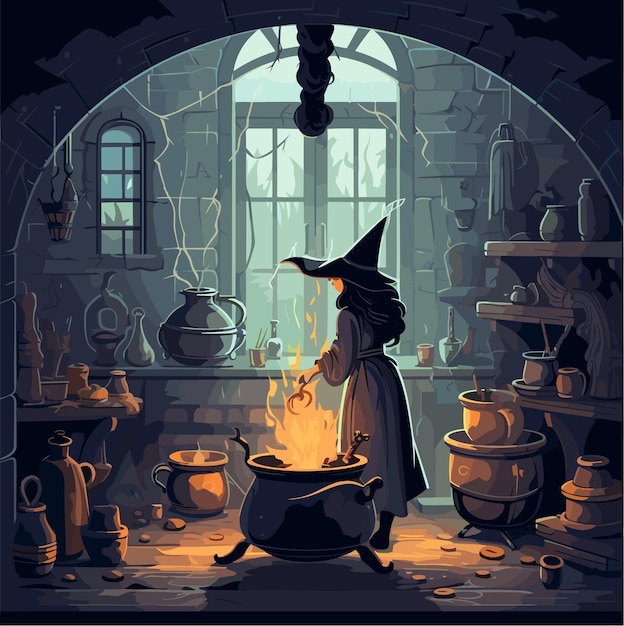The image is a digitally created cartoon-like depiction of a young witch in her shadowy workshop, meticulously adorned with a classic black, pointy witch's hat and a gray dress. She stands with her back to the viewer, her long dark hair cascading down, as she tends to a large, central cauldron from which fire emerges, casting a warm, orange glow on her surroundings. The cauldron appears to be part of a spell or potion-making process, as her hand hovers above it, dropping either a bone or an apple into the flames – the exact object remains unclear.

Her mysterious workshop, predominantly shrouded in black, white, and greenish-gray hues, is visibly illuminated by the soft light filtering through a large window at the back, which offers a glimpse of the outside. This light also reveals numerous details inside the dimly lit room, including cobwebs and various vases and jars scattered around. Shelves, placed to the right of the witch, hold various uncapped glass containers, while a table to the left and another counter at the rear display a range of potion ingredients in jars, some sealed and some open.

Additional elements like a bucket filled with unlit candles in the upper left corner and small white streaks through the image hint at the presence of either spider webs or some form of magical energy, adding to the enchanted, eerie atmosphere of the scene.